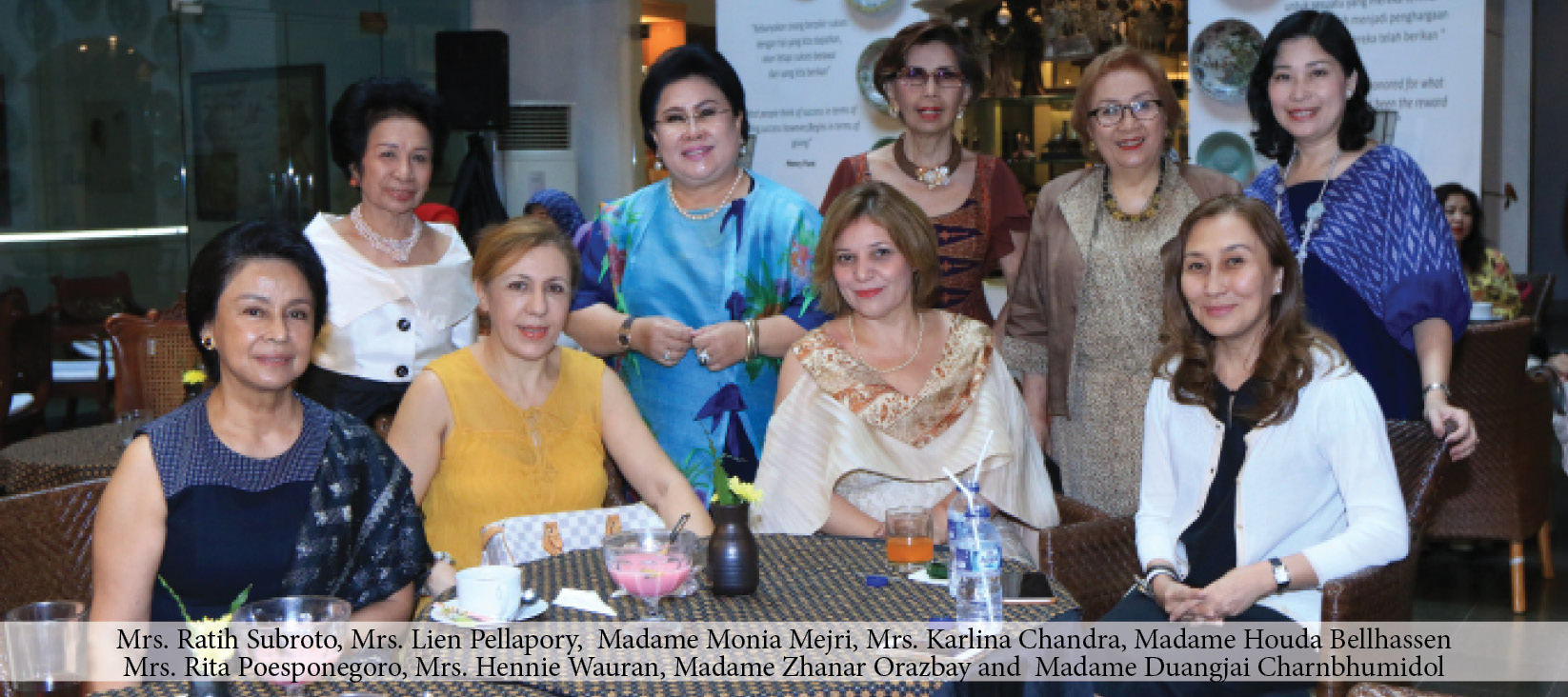A wide-angle group photograph captures nine women, seemingly in their 40s or older, dressed for a special event. In the foreground, four women are seated around a table adorned with a yellow and blue checkered tablecloth, featuring various drinks including a flower-adorned beverage, a bowl with pink liquid, and a cup of coffee. From left to right, the seated women include an elderly woman in a blue dress with black hair, a woman with blondish hair in a yellow blouse, another with a shawl around her shoulders, and one in a white sweater. Behind them, five more women stand, all smiling warmly at the camera. A solitary woman can also be seen in the distant background, seated at another table. At the bottom of the photo, a white border displays the names of all nine women in black text: Ms. Rati Sobroto, Ms. Lian Palapuri, Madam Monia Majuri, Ms. Carlina Chandra, Madam Huda Belhassan, Ms. Rita Pospinagoro, Ms. Hennie Warren, Madam Zanara Orozbay, and Madam Tungjai Charnbomidal. The exact order of the names relative to the positions of the women in the photo is uncertain.